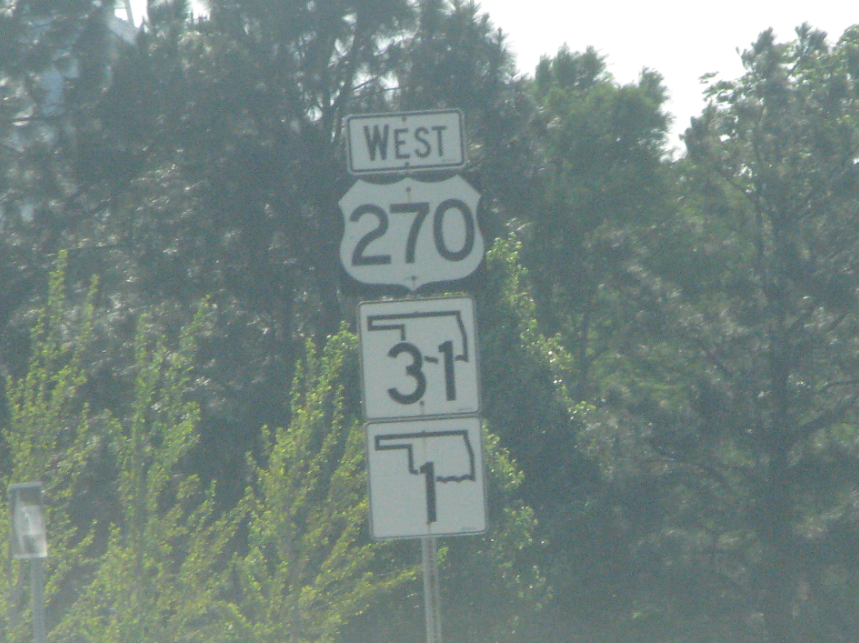A close-up photograph captures a series of four road signs mounted on a single round silver pole, set against a backdrop of dense trees. At the top of the pole is a small rectangular sign indicating "West." Below it, a square sign features the number "270" within a white square bordered in black. The third sign displays the outline of the state of Oklahoma with the number "31" overlaid on it. The fourth and final sign, similar in design, shows the outline of Oklahoma with the number "1." In the top right corner of the image, the trees give way to a brighter, light-filled sky. Additionally, between the trees on the right side, there is a discernible outline of what appears to be the top of a mountain.